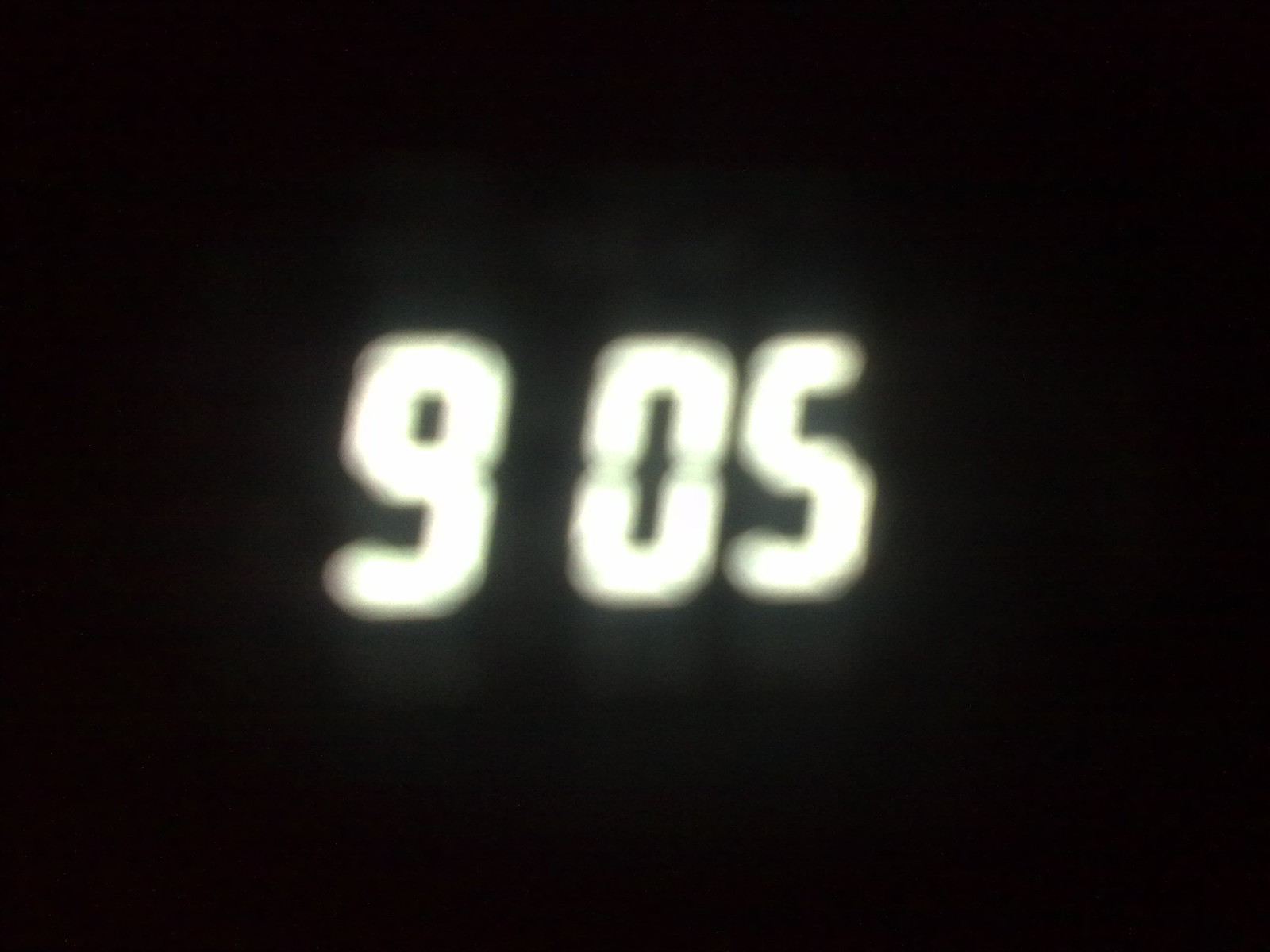A minimalist digital clock face showing the time "9:05" stands out vividly against a completely black background. The numerals, illuminated with an intense and radiant white glow, are so bright that the usual line breaks between the segments of the digits are mostly obscured, except for the two discernible breaks within the "0". This powerful luminosity gives the numerals an almost seamless appearance, creating a striking contrast with the pitch-dark surroundings. The overall effect is a stark, almost ethereal depiction of time in its simplest digital form.